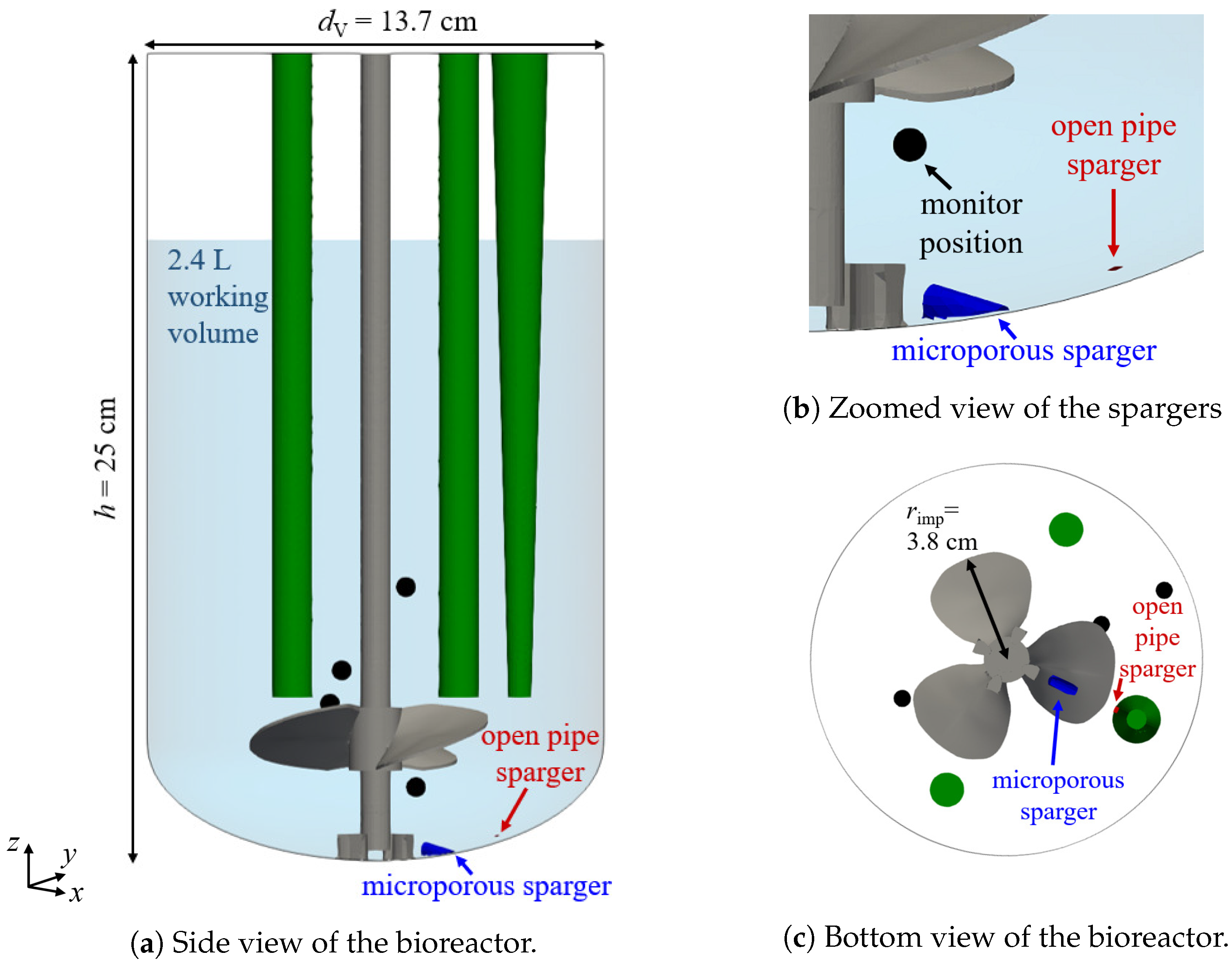This detailed diagram depicts various views of a bioreactor setup with specific dimensions and features. On the left side, the side view of the bioreactor shows a cylindrical tank containing a blue liquid, indicating a working volume of 2.4 liters. The tank measures 25 centimeters in height and 13.7 centimeters in depth. Inside the tank, there's a gray turbine-like structure, with green rods that extend vertically to the top of the tank. 

At the bottom of the side view, two types of spargers are labeled: "open pipe sparger" and "microporous sparger." The right side of the diagram provides additional insets. The top inset (labeled B) offers a zoomed view near the turbine, pinpointing the position of the monitor and the open pipe sparger. The bottom right inset (labeled C) presents an overhead view of the bioreactor. This inset clearly shows the circular arrangement of the turbine fan along with the positions of the spargers and green dots representing the pipes. The diagram also indicates the dimension of the impeller radius (r imp) as 3.8 centimeters, contributing to a comprehensive understanding of the bioreactor's layout.